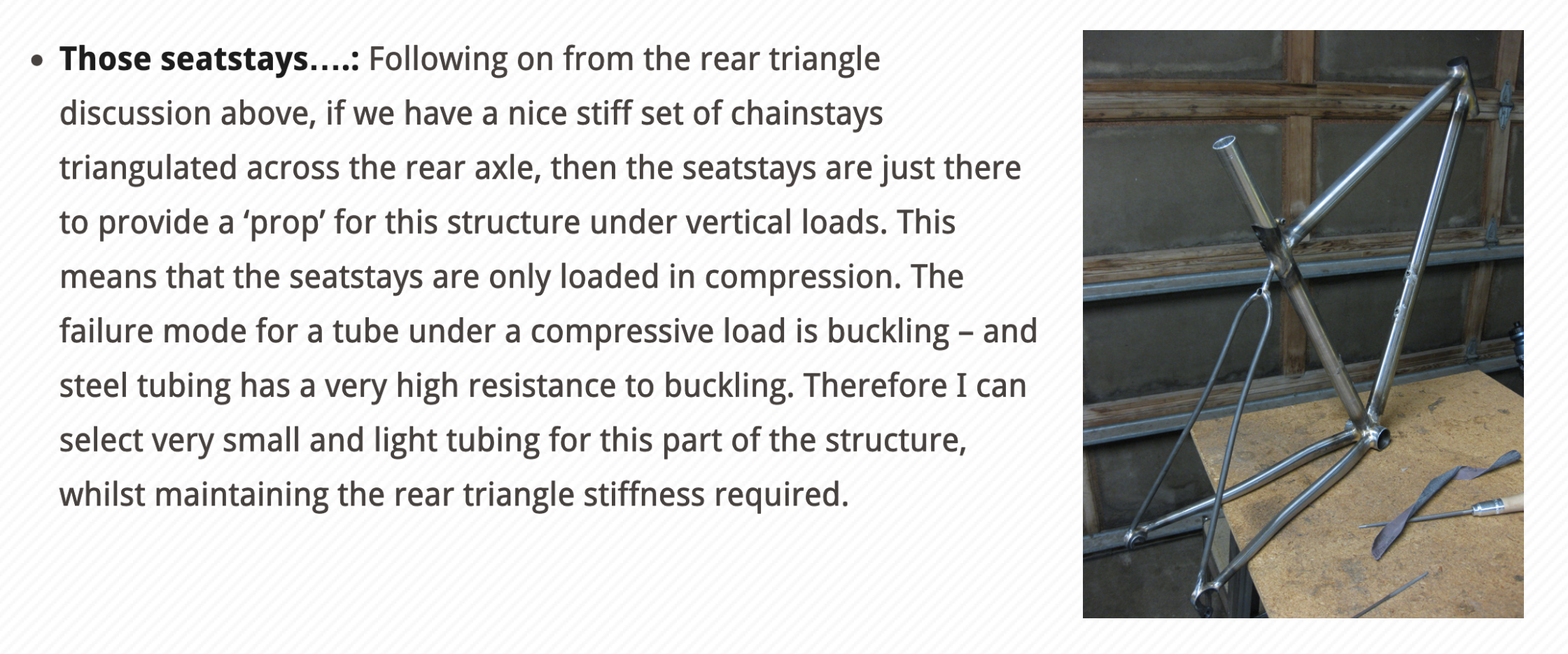The image depicts a metal structure resembling a hammock support system, composed of a metal base with two legs and an arm extending to the right. Set against a white background, the image includes bold black text stating, "those seat stays." The text details the mechanical function of the seat stays following a discussion of the rear triangle above. It explains that with a stiff set of chainstays triangulated across the rear axle, the seat stays merely prop up the structure under vertical loads, operating in compression. Steel tubing is noted for its high resistance to buckling, allowing the use of small, lightweight tubing while maintaining the required stiffness of the rear triangle. The metal structure, positioned on a wooden table, appears to be under construction, likely in a garage setting, with a closed garage door and well-lit surroundings visible in the background.